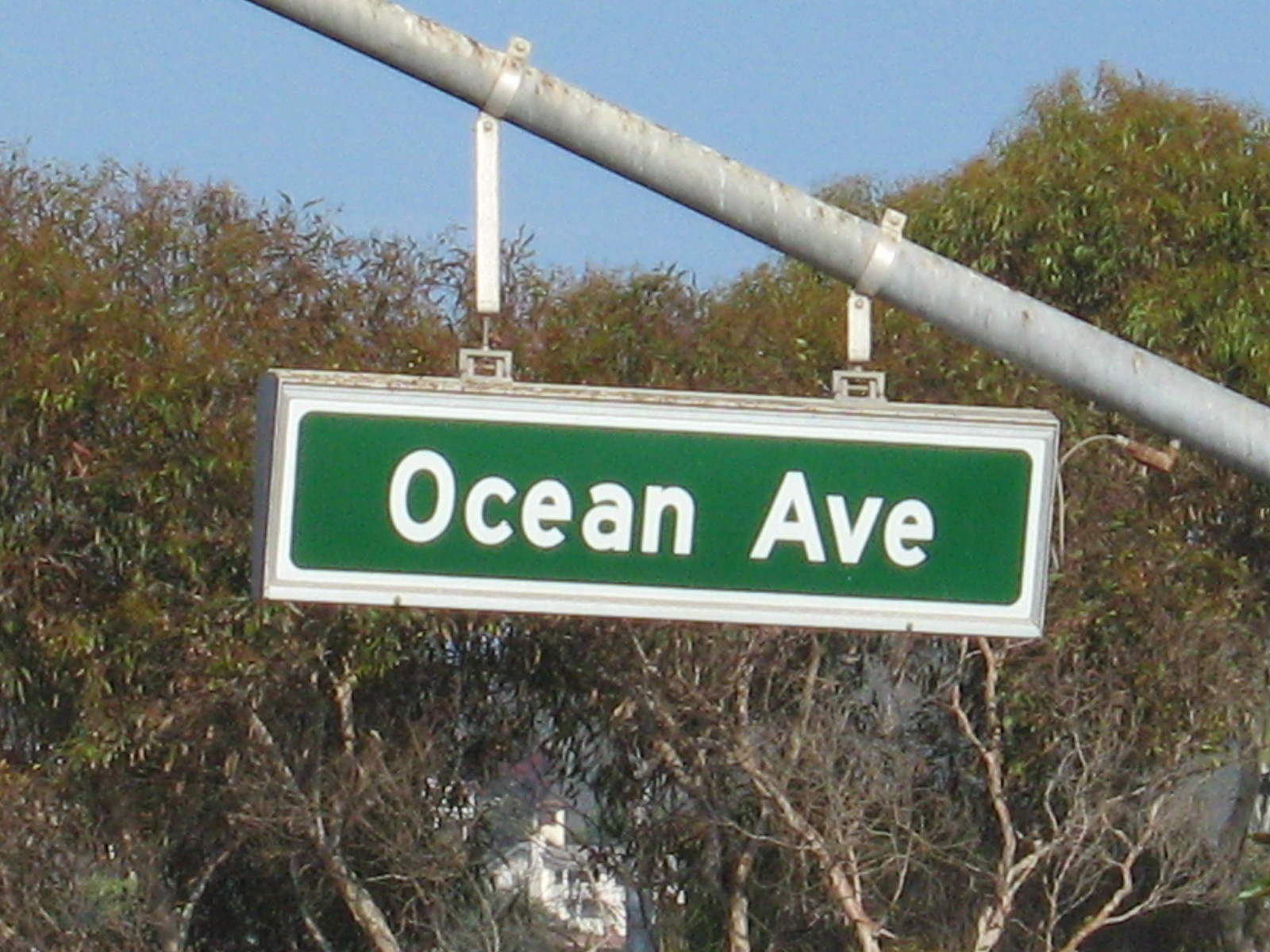A street sign for "Ocean Avenue" is prominently displayed, suspended from an angled metal pole. The pole, which diverges from the conventional vertical orientation, is fixed at an approximate 30-degree angle across the roadway. Supporting this unique setup are metal straps of varying lengths, reminiscent of those used to secure piping. The sign itself features a green background with crisp white lettering, ensuring high visibility. In the background, a dense cluster of coastal shrubs and trees, with matted and interwoven branches, reaches a height of three to four feet. Nestled beneath this verdant foliage and slightly in the distance, a white house or structure is partially visible, adding a touch of architectural contrast to the natural scene.